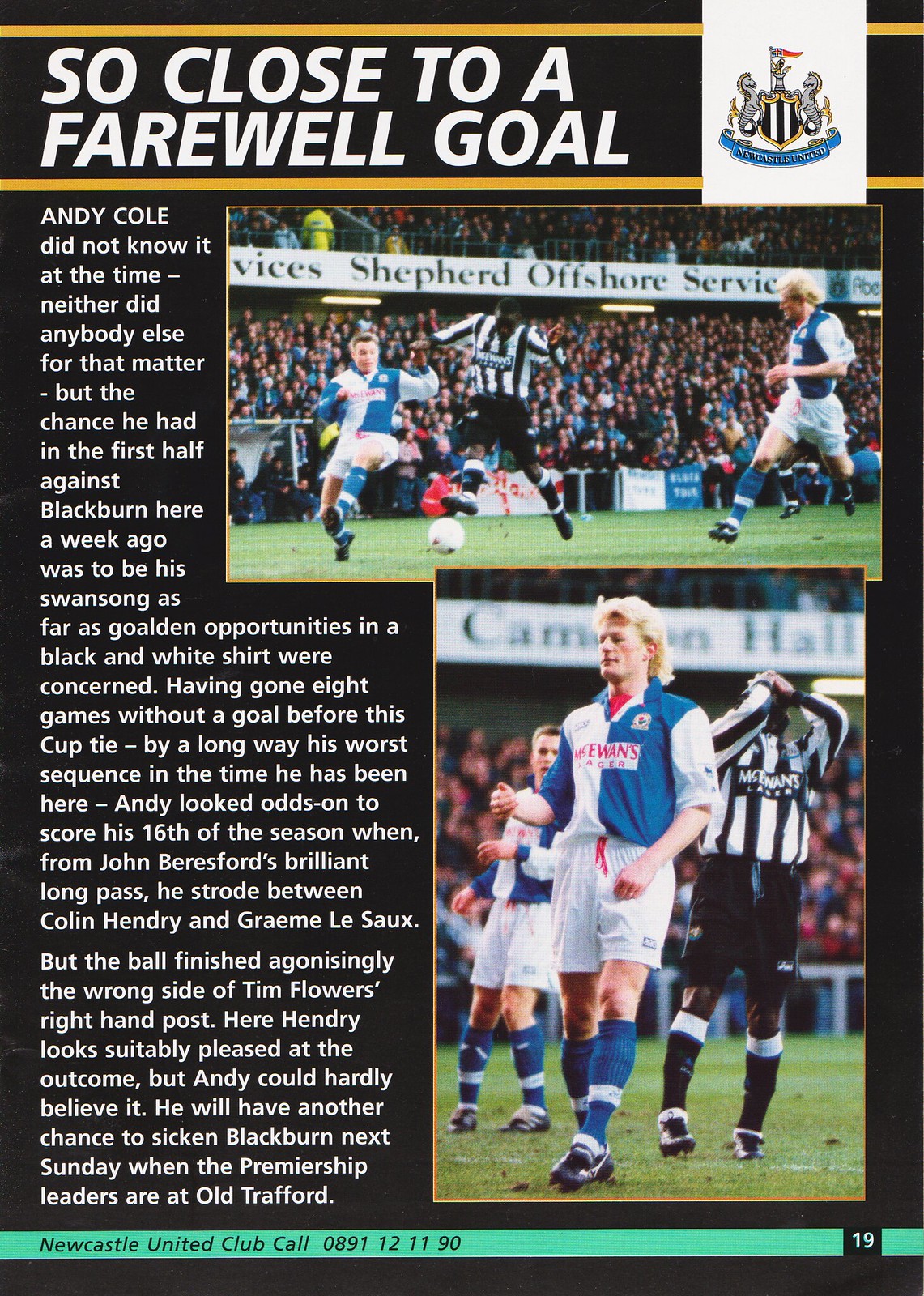The image resembles a page from a magazine or book about soccer, featuring a black background that creates a striking contrast. At the top, in white text, the title reads "So Close to a Farewell Goal," framed by golden yellow horizontal bars above and below. To the right of the title is the Newcastle United Football Club logo on a white rectangle.

On the left side, a comprehensive paragraph of white writing mentions Andy Cole, identifying him as the subject. It describes how neither he nor anyone else knew that a recent chance against Blackburn would be one of his last significant goal opportunities in a black and white shirt.

Occupying the right two-thirds of the image are two photographs from a soccer match. The top photo shows Andy Cole, a black player in action, kicking a ball while two opponents in white and blue jerseys pursue him. The bottom photograph features a tense moment with a white player, blonde and wearing a blue and white jersey, standing mid-field, while behind him, Andy Cole, hands on his head, displays frustration in his Newcastle United kit of black and white stripes. Below this, a blue-green stripe runs horizontally with the text "Newcastle United Club call 0891 121190" in black, and a black square with the number "19" in white is situated on the stripe's right side.